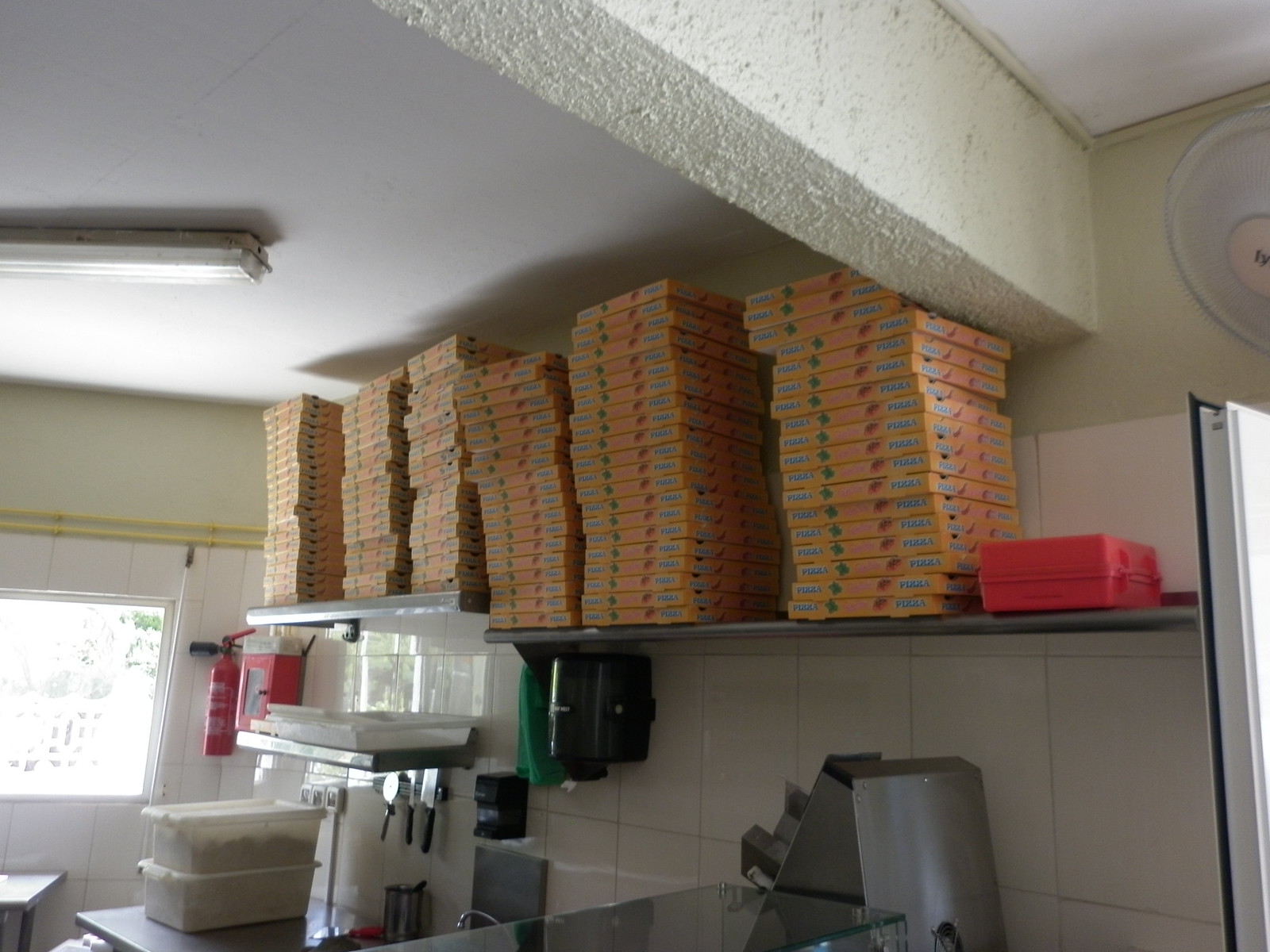This image appears to be taken inside a pizza restaurant, focusing on the upper portion of a kitchen wall covered in white ceramic tiles. On the left side of the image, there's a window revealing a bright exterior. Just to the right of the window, you can see a fire extinguisher mounted on the wall. Below the window rests a counter where two Tupperware boxes are stacked on top of each other. Above this counter, two metallic shelves are installed; the left shelf is slightly higher and less wide compared to the right. Both shelves each have three rows of identical pizza boxes stacked on them. Notably, at the far right end of the right shelf, there's a red plastic box resembling a lunch box. Overhead, a fan is visible in the upper corner, and various kitchen utensils including knives, as well as a green item, are affixed to the wall. The bottom half of the image shows what appears to be a sliver of silver kitchen machinery.